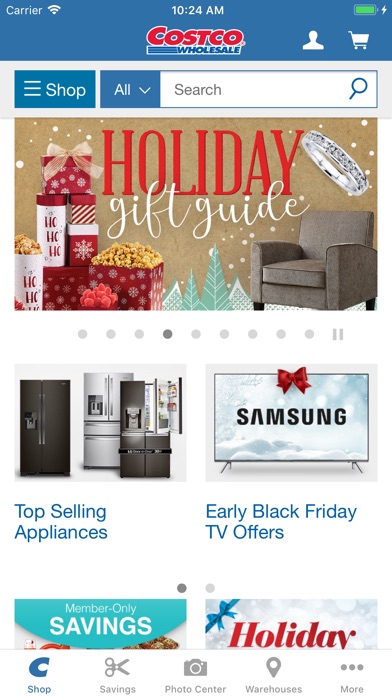Screenshot of a mobile device displaying the Costco homepage:

At the top, a header with a blue background prominently features the red Costco logo. Below the header, a navigation bar consists of a gray rectangle with two blue tabs. The first tab, marked by three horizontal lines, is labeled "Shop." The second tab, positioned adjacent to a white search bar, is labeled "All." The search bar contains the text "Search" and is accompanied by a magnifying glass icon.

The main section of the page features various promotional content. A large rectangle titled "Holiday Gift Guide" displays an assortment of festive items, including a red square box adorned with white snowflakes containing popcorn. Several other gifts surround the box—some wrapped, others open revealing various snacks. Small Christmas trees decorate the bottom of the image, while a black-gray chair sits to the right. Above this chair is an enlarged illustration of a wedding ring.

Below this promotional content, a series of pagination dots indicates multiple pages of content are viewable. The next section highlights two more offers. The first, "Top Selling Appliances," showcases three refrigerators: two black and one gray, with the gray refrigerator positioned in the center. The second offer, "Early Black Friday TV Offer," features a Samsung TV topped with a red bow. The TV screen displays a winter scene with falling snow, snowflakes, and a snowy tree.

At the bottom of the screen, two partially visible sections are labeled "Member Only Savings" and "Holiday," although their full content is cut off. The footer navigation menu spans the width of the screen with five clickable icons: "Shop," "Savings," "Photo Center," "Warehouses," and "More," each accompanied by corresponding icons.

The overall design is festive and geared towards holiday promotions, with a mix of cheerful graphics and practical product offerings.